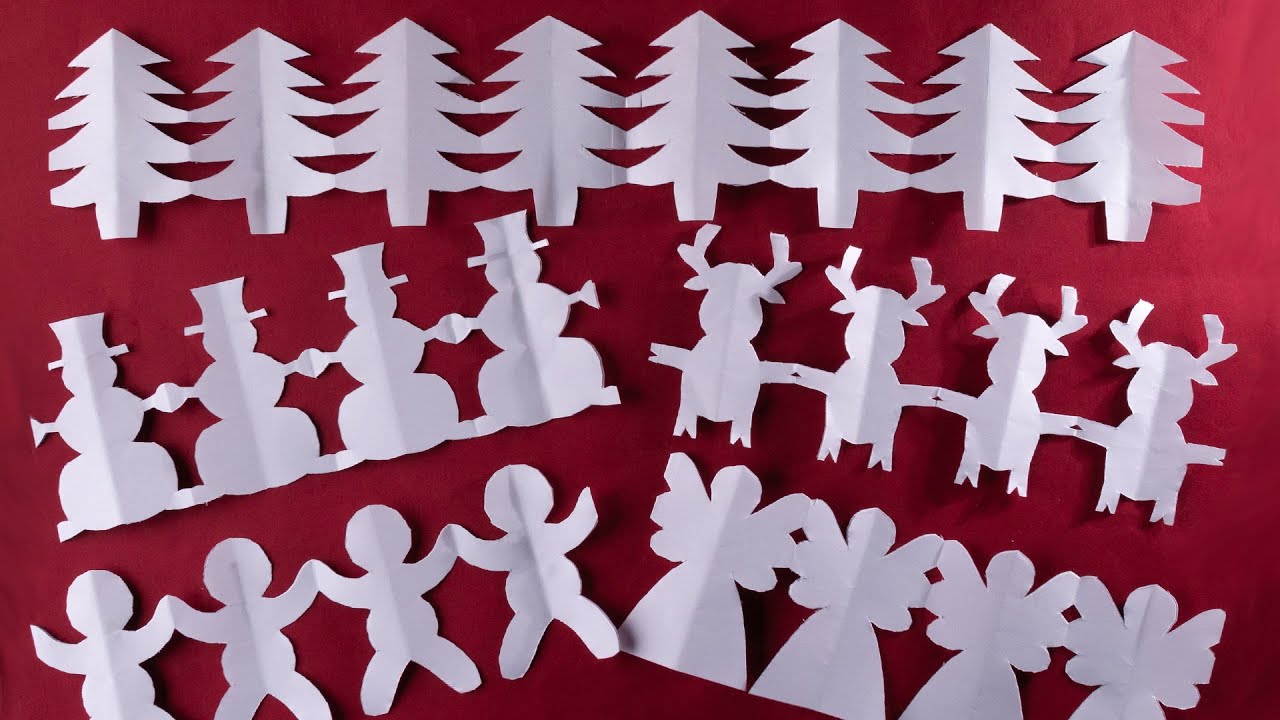This is a detailed image featuring an assortment of white paper cutouts intricately arranged on a rich red background. At the top, there is a row of eight paper cutout pine trees, forming a festive, forest-like border. Along the left side of the image, there is a vertical series of paper cutouts, starting with four snowmen positioned in the middle left, followed by four human-like figures or possibly gingerbread men below them. On the right middle section, four reindeer are neatly aligned, adding to the holiday theme. The bottom right corner features a row of four angels. All cutouts are connected in a chain-like fashion typical of folded and cut paper crafts, enhancing the overall Christmas ambiance of the image.